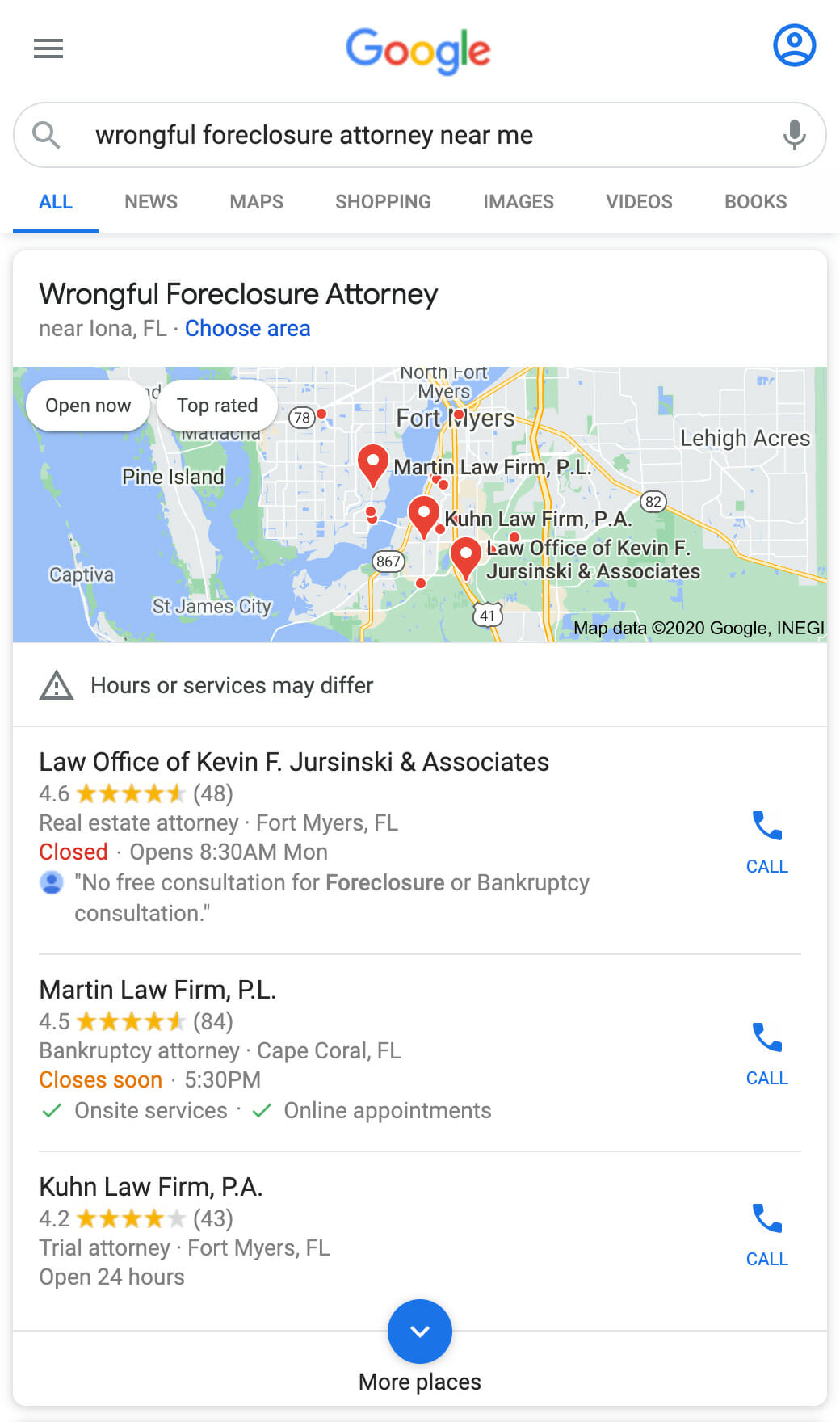A screenshot of a Google search on a mobile device displays the familiar Google logo at the top, with the two 'G's in blue, the 'O' and the 'E' in red, the second 'O' in yellow, and the 'L' in green. On the left side, a three-horizontal-lines menu dropdown icon is visible, and on the right, a blue circle featuring a person icon represents the user's profile. 

Below the logo, the search bar contains the query "wrongful foreclosure attorney near me," flanked by an eyeglass icon on the left and a microphone icon on the right. Under the search bar, there are several tabs labeled: All, News, Maps, Shopping, Images, Video, and Books, with the "All" tab selected.

Further down, a large white rectangle displays the update "wrongful foreclosure attorney near Iona, Florida," accompanied by a blue text option to "choose area." Beneath this text, a map of Iona, Florida highlights various law offices with markers and pins. 

Three major entries are featured prominently on the map:

1. **The Law Office of Kevin F. Jurinski and Associates** 
   - Real estate attorney in Fort Myers, Florida 
   - Rated 4.6 out of 5 stars
   - Does not offer free consultations for foreclosure or bankruptcy.

2. **Martin Law P.L.**
   - Bankruptcy attorney in Cape Coral, Florida
   - Rated 4.5 out of 5 stars
   - Closes soon at 5:30 p.m.
   - Provides on-site services and online appointments.

3. **Kuhn Law Firm P.A.**
   - Trial attorney in Fort Myers, Florida
   - Rated 4.2 out of 5 stars
   - Open 24 hours.

To the right of each entry, there's a blue phone icon accompanied by the word "Call" in blue text, allowing users to contact the listed law firms directly.